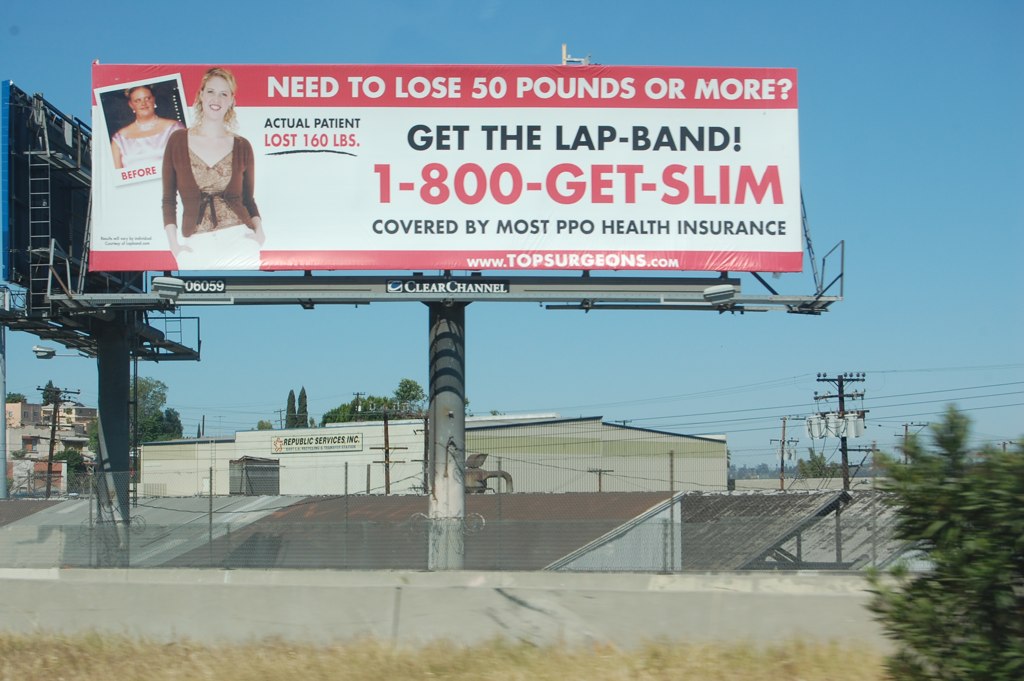This color photograph captures an industrial scene dominated by a large billboard mounted on a silver cylindrical pole near the center of the image. The foreground features a stretch of dry, brownish-yellow grass and a sizable green tree that extends about a third of the way up on the right side. Just behind the grass and tree, a concrete barrier runs horizontally across the scene, topped by a chain-link fence.

The billboard, prominently positioned above the barrier, has a striking red border with a white center. At the top, the text reads, "Need to Lose 50 Pounds or More," and below it in bold, it says, "Get the Lap Band!" with a number, "1-800-GET-SLIM," in red. Further down, it states, "Covered by Most PPO Health Insurance" and lists the website "www.topsurgeons.com," all in black text. The advertisement also includes images of a woman, with a caption indicating she lost 160 pounds, highlighted by different color fonts for emphasis.

Behind the barrier, a mix of industrial buildings with worn red and black roofs can be glimpsed, and to their side, a larger beige building displaying a sign for "Republic Services." The background reveals power lines and poles under a clear blue sky, framing the entire scene.